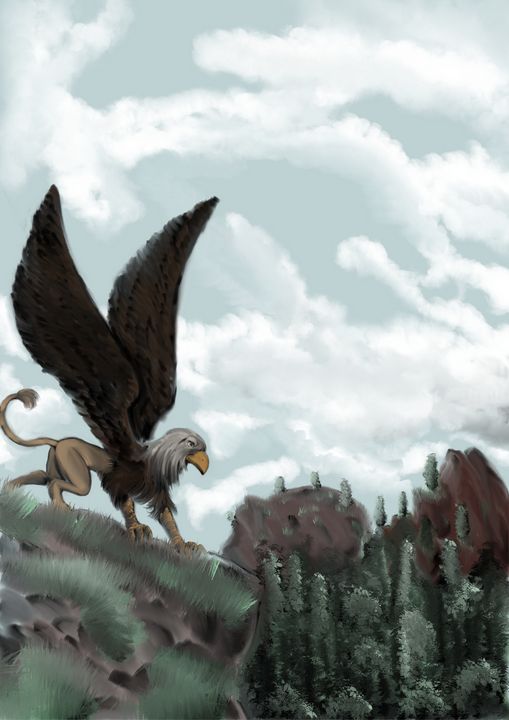This detailed digital painting portrays a majestic griffin perched on a hillside, surveying a diverse landscape. The griffin, a mythical creature with the head and wings of a bald eagle and the body of a lion, is depicted with striking realism. Its vivid orange beak and large, brown wings are prominent features. The hillside beneath the griffin is covered in short green grass, interspersed with black rocks. To the right of the creature, the terrain transitions into a desert landscape dotted with green cactuses, while in the distance, the scene is framed by brown mountains. The sky above is filled with wispy white clouds against a light blue backdrop, creating a serene yet dramatic atmosphere. The griffin’s lion-like paws and bushy tail are visible as it stands firmly on all fours, embodying both strength and grace. The overall scene is a harmonious blend of verdant forests, rugged desert, and towering mountains, all unified under a tranquil, cloud-filled sky.